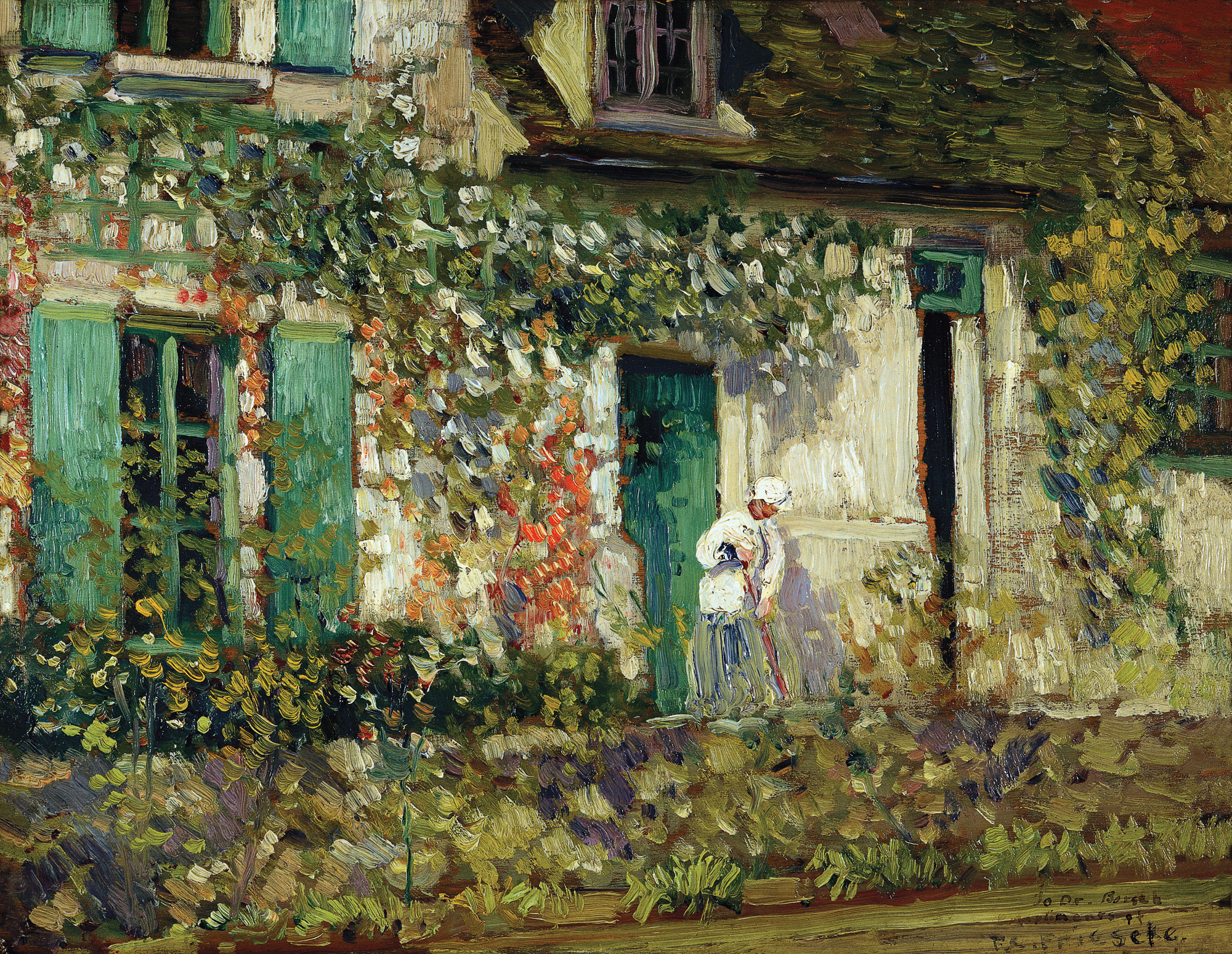This painting, reminiscent of Monet's impressionist style, captures a bucolic scene of an old country house enveloped by lush greenery and vibrant flowers. The two-story house, painted in white, features mint green window panes and shutters, and a green front door, partially obscured by ivy and vegetation, which may also extend onto the greenish roof. A notable feature is the woman positioned just right of center, with dark brown skin, engaged in sweeping the front steps. She is dressed in a white bonnet, a white long-sleeve top, and a dress/skirt that transitions into shades of blue and green at the bottom. The foreground is richly adorned with a variety of plants and flowers, including hues of white, purple, orange, and coral, creating a vivid, nature-filled setting. The composition is highlighted with additional accent colors such as black, brown, pink, and red. The artist's signature, although illegible, is scrawled in the bottom right-hand corner, completing this captivating impressionist scene.